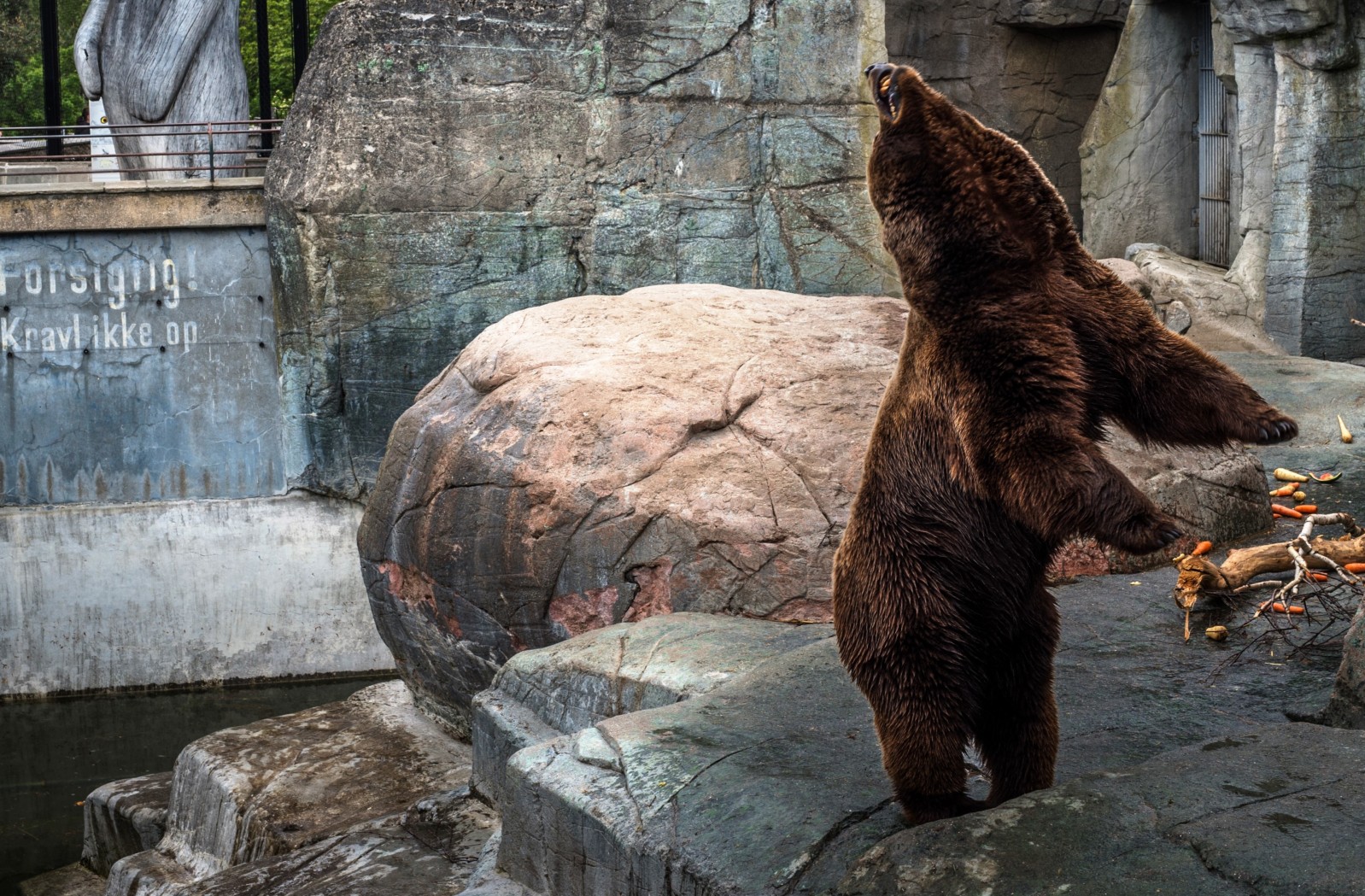This photograph, taken at a zoo, features the main attraction: a large, dark brown grizzly bear. The bear is poised on its hind legs atop a mound of dark, granite-like rocks with shades of black and gray. Its front legs are outstretched, and it appears to have its head reared back, either looking up or preparing to catch something, perhaps food thrown by a zookeeper. The enclosure, surrounded by big brick walls in gray and blue tones, also includes other rock formations and a scattered branch. A vantage point for visitors can be seen in the background beyond a small fence, along with a body of water near the ground, providing a naturalistic habitat for the bear. The bear's powerful stance and open mouth suggest it might be roaring or anticipating a treat, adding drama to the scene. The floor of the enclosure is littered with small branches and possibly scattered carrots, enhancing the realistic, rugged environment.